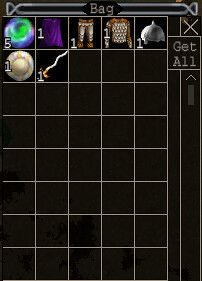This image is a detailed screenshot from a game, showcasing the green user interface, specifically the inventory section. The top of the screen features the word "Bag" inside a black diamond shape with grey letters. To the top right, there's a "Get All" button in white text on a grey vertical slide. The inventory layout consists of a black background with white horizontal and vertical lines forming a grid of columns and rows. Each grid slot displays various items. Notably, there is a multi-colored bowl marked with the number 5, a purple cape with the number 1, a white and gold shirt also labeled with the number 1, a piece of armor and a helmet each bearing the number 1, and a sword with a gold handle and silver blade, similarly marked with the number 1.